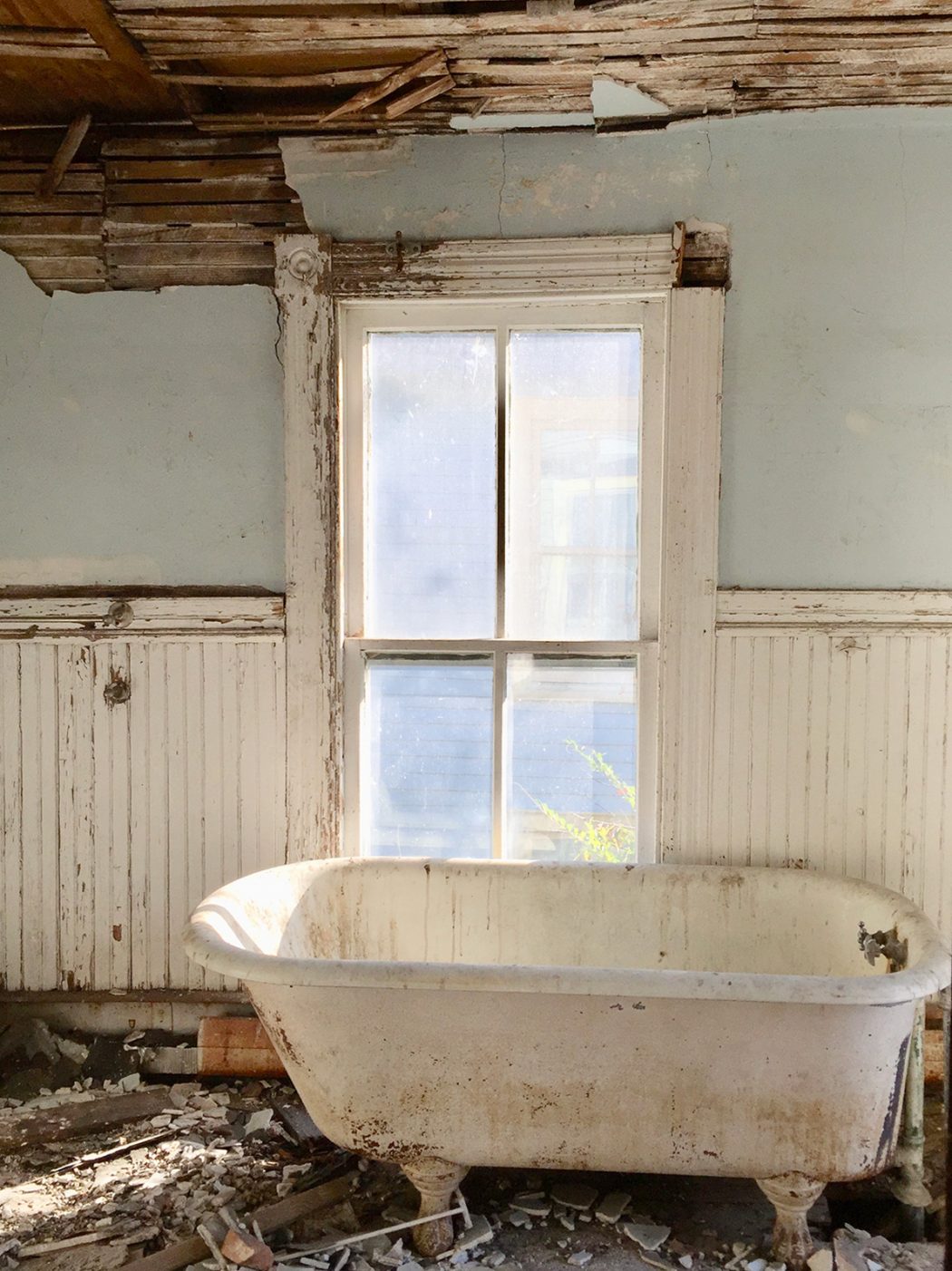The photograph depicts a severely dilapidated bathroom that appears to have endured significant damage, possibly from a storm. At the center of the image is a filthy, white claw-footed bathtub positioned on a floor strewn with broken drywall, tiles, glass, and other debris. The tub's exterior is heavily stained, with faucets located on its right side. Surrounding the tub, the wall features a bottom half covered in shiplap paneling painted white but now peeling significantly. Above this, the wall is painted light blue, though much of the paint has deteriorated, exposing the wooden paneling beneath. Directly above the bathtub hangs a large four-panel window, its frame also white and peeling, offering a glimpse of daylight and a small plant outside. The chaos continues to the ceiling, where wooden slats hang precariously, contributing more debris to the mess below. This once functional bathroom now stands in a state of utter disrepair and neglect.